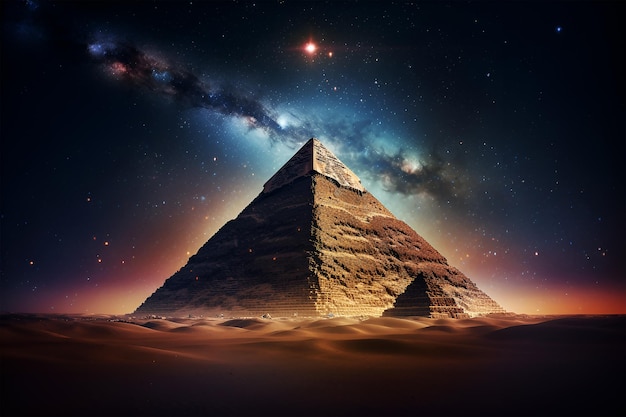This digital image vividly captures a nighttime desert scene featuring a prominent brown pyramid with a smaller pyramid in front of it to the right. The larger pyramid shows brownish-gray hues and fading facades, leaving a clearer top. Surrounding the pyramids, the sand-covered ground transitions to black towards the bottom.

The sky in the background is a deep navy blue, punctuated by a scattering of stars, with a particularly bright red star at the top, distinguished by a white center. Hints of teal and black add depth to the dark night sky, and a nebula stretches diagonally behind the pyramid. The image is saturated with various colors, including oranges, tans, blues, blacks, whites, and grays. The scene is further accentuated by a reddish, pinkish glow around the pyramid, complemented by illuminating lights that resemble fiery flames. Overall, this richly colored and detailed image combines elements of both natural and celestial beauty.